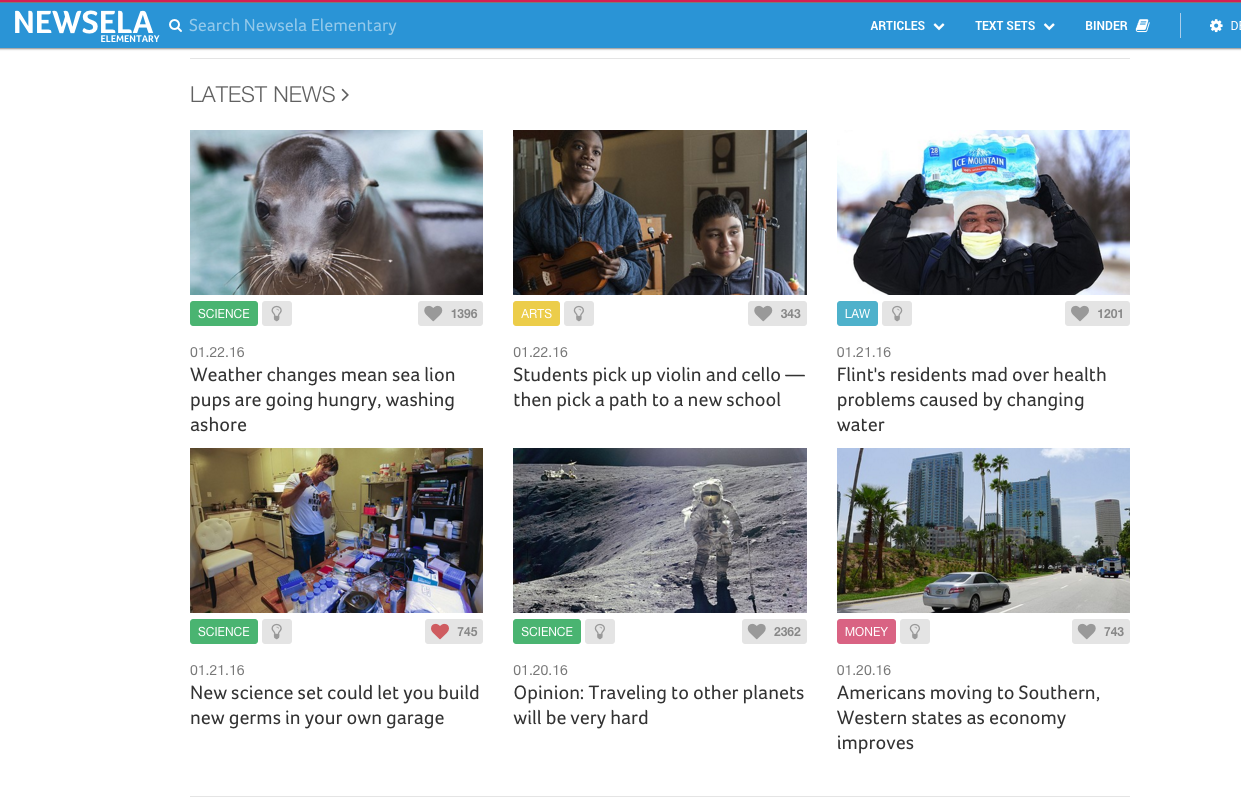Screenshot of the New Silla Elementary Website with Articles Overview

The screenshot showcases the New Silla Elementary website, featuring a prominent blue banner. Positioned at the top left corner is the New Silla Elementary logo. Adjacent to the logo is a search bar, while the far right of the same row includes tabs for "Articles," "Text Sets," "Binder," and "Settings." The top edge of the header is outlined in red, the only red element on the page.

Below the header, the main content area displays four highlighted articles under the section labeled "Latest News," each accompanied by images. Detailed descriptions of the first two articles are as follows:
1. The first article, titled "Weather Changes Mean Sea Lion Pups Are Going Hungry, Washing Ashore," reports on environmental impacts affecting sea lions. It was posted on January 22, 2018, and features a "Science" tag beneath its photo. The article has garnered 1,396 likes, indicated by a heart icon, and is also marked with a lightbulb icon, which likely denotes an educational focus.

2. The second article, "Students Pick Up Violin and Cello, Then Pick a Path to a New School," was also published on January 22, 2018. It bears "Arts" and "Lightbulb" tags and has received 343 likes. The accompanying image features two male students; one holds a wind instrument while the other holds a cello. 

The entire website background is white, providing a clean and structured layout for presenting the educational content.